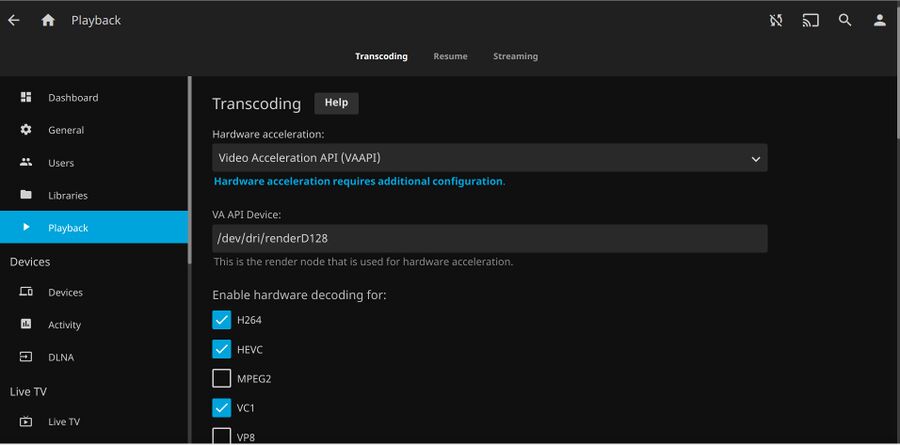The image captures a user interface with a predominantly black background, detailing various options and information. In the top left corner, there's a white arrow pointing left next to the text "Play Back" in white. Accompanying this are several icons, including a search icon and two arrows pointing in different directions, potentially signifying navigation or synchronization. There's also a box icon commonly associated with Wi-Fi. In the center, bold white text reads "Transcoded" with "Resume Streaming" in regular white text beneath it.

On the left side of the interface, a navigation menu is displayed in white text. The options listed, from top to bottom, are:

- Dashboard
- General
- Users
- Libraries

The "Play Back" section is highlighted in blue, followed by:

- Devices
- Devices Activity
- DLNA
- Live TV (repeated twice)

Further down, a partially visible section mentions "transcoded" again.

To the right, a gray box titled "Help" contains text about hardware acceleration. Inside this box, the text reads: 
"Hardware acceleration requires additional configuration."

Below this, another gray box specifies:
"Video Acceleration API (V-A-A-P-I)." 

Following some space, white text outlines configuration details:
"V-A-A-P-I device: /dev/dri/renderD128. This is a render code used for hardware acceleration."

Additional instructions advise enabling hardware decoding for formats including H264, HEVC, MPEG-2, VC-1, and VP8.